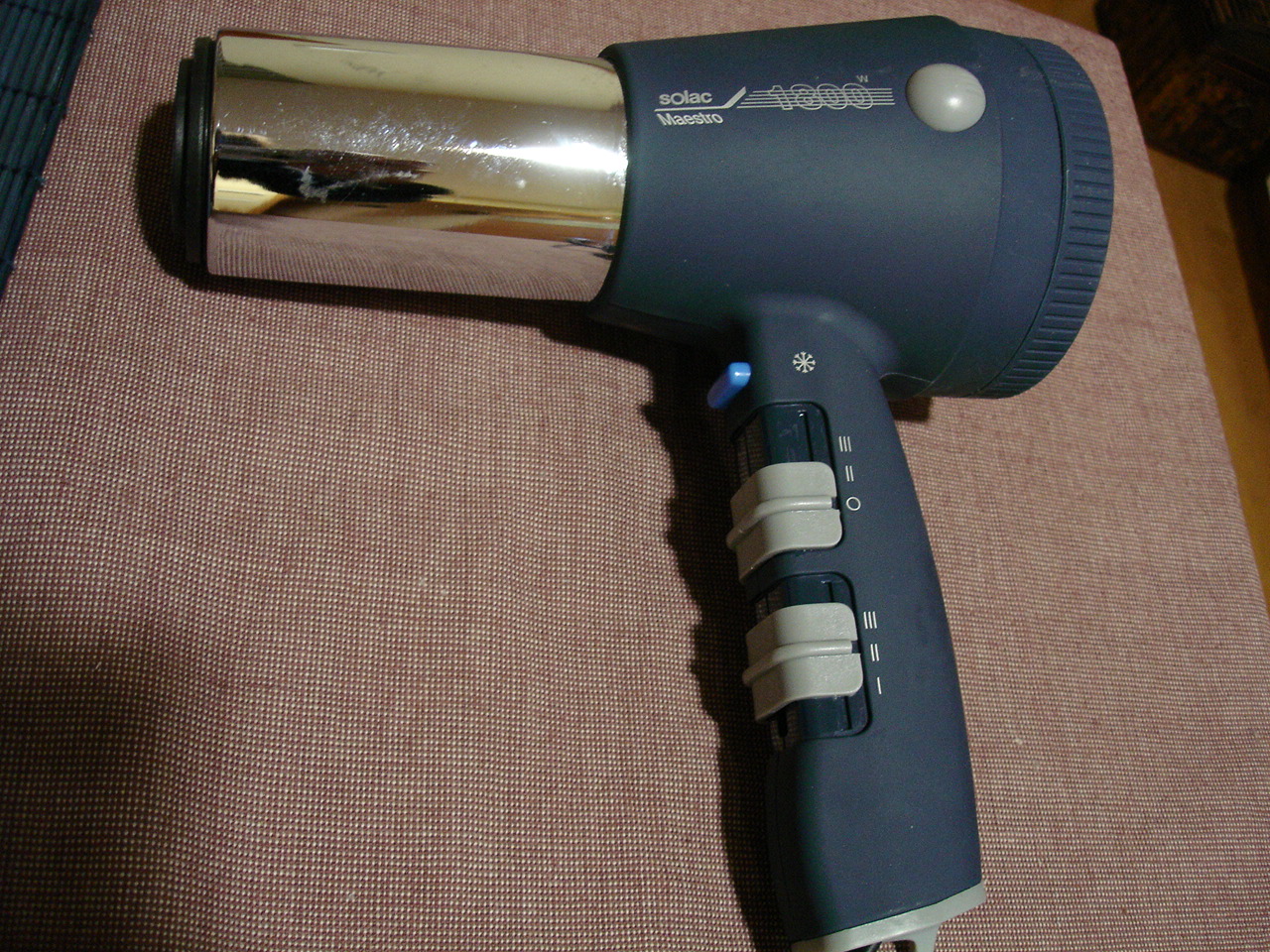This image showcases a vintage hairdryer laying on a pink textile with a grid-like pattern of white and amber colored threads. The hairdryer features a chrome-colored cylindrical shaft pointing to the left, adorned with a bright red reflection and noticeable scratches. The main body of the hairdryer, a dark blue color, displays "Solac Maestro 1800" in light gray letters, accompanied by a line underneath. To the right of the text are several horizontal lines and a gray circular button. The handle, also blue, houses a light blue button reminiscent of a snowflake, presumably for a cooling function, and gray adjustable knobs marked with various symbols—circles and lines indicating different settings. The hairdryer appears to rest atop a medium brown wood-colored counter, adding a rustic element to its vintage design.